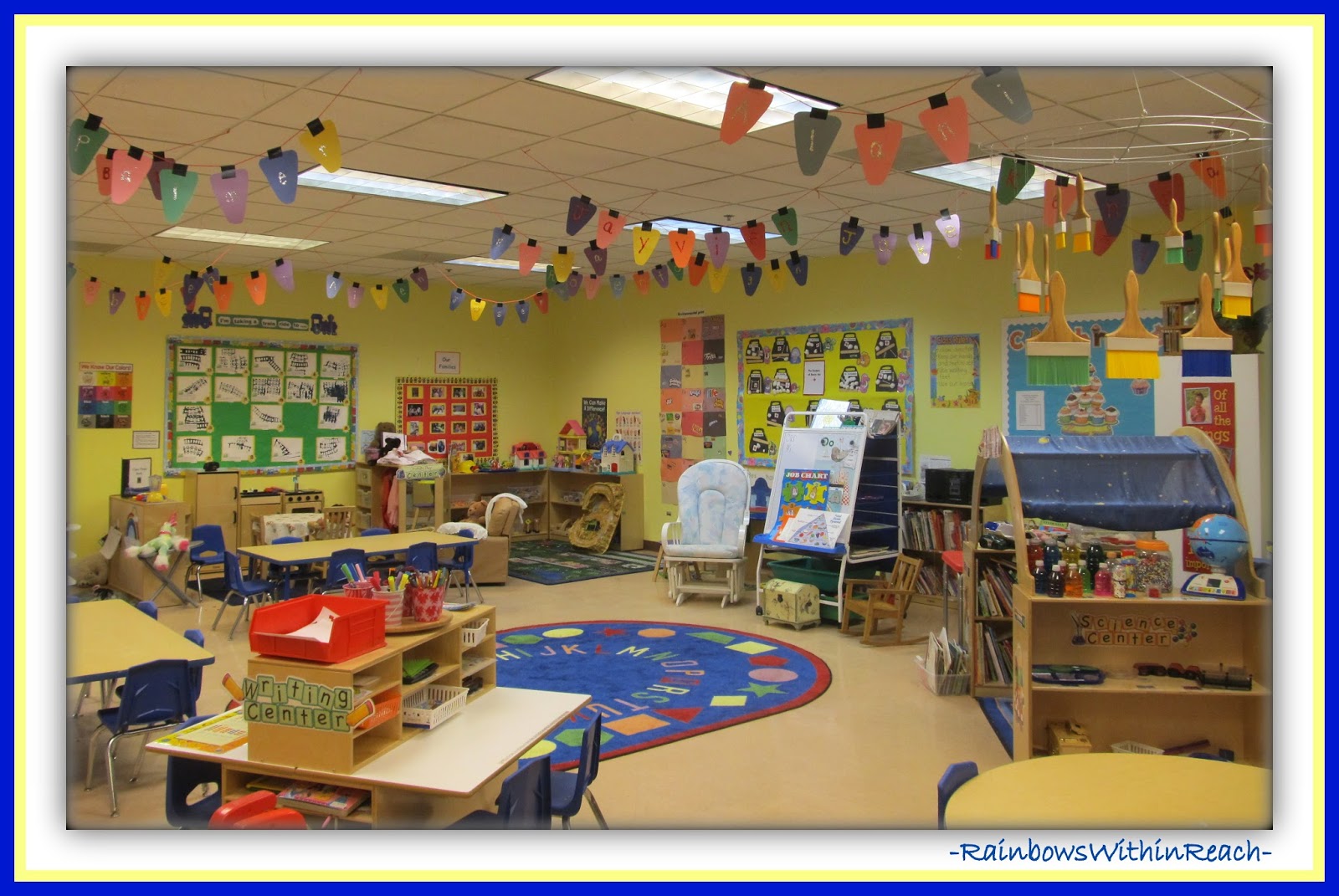The image depicts a vibrant and bustling preschool or kindergarten classroom, designed to inspire and engage young minds. The space features yellow walls adorned with several bulletin boards filled with children's art and educational materials. A prominent green bulletin board alongside a smaller red one is covered with colorful drawings. Children's size desks and chairs are arranged alongside these walls, and an inviting blue rug with a red border, themed with the alphabet, lies in the center of the room. The rug is surrounded by more desks and marks out a designated area that includes a writing center, identified by a divider and four chairs.

The room's ceiling is a drop style with fluorescent lights, further brightened by various hanging mobiles and jumbo Christmas light-shaped items. Paintbrushes, arranged in a beautiful spiral pattern, dangle in cheerful bursts of color. A rocker recliner adds a cozy seating option. Storage areas, art supplies, and other educational materials are strategically placed around the classroom, enhancing its function and charm. Notably, the words "rainbows within reach" are inscribed in blue letters at the bottom right, reflecting the room's imaginative and welcoming atmosphere.